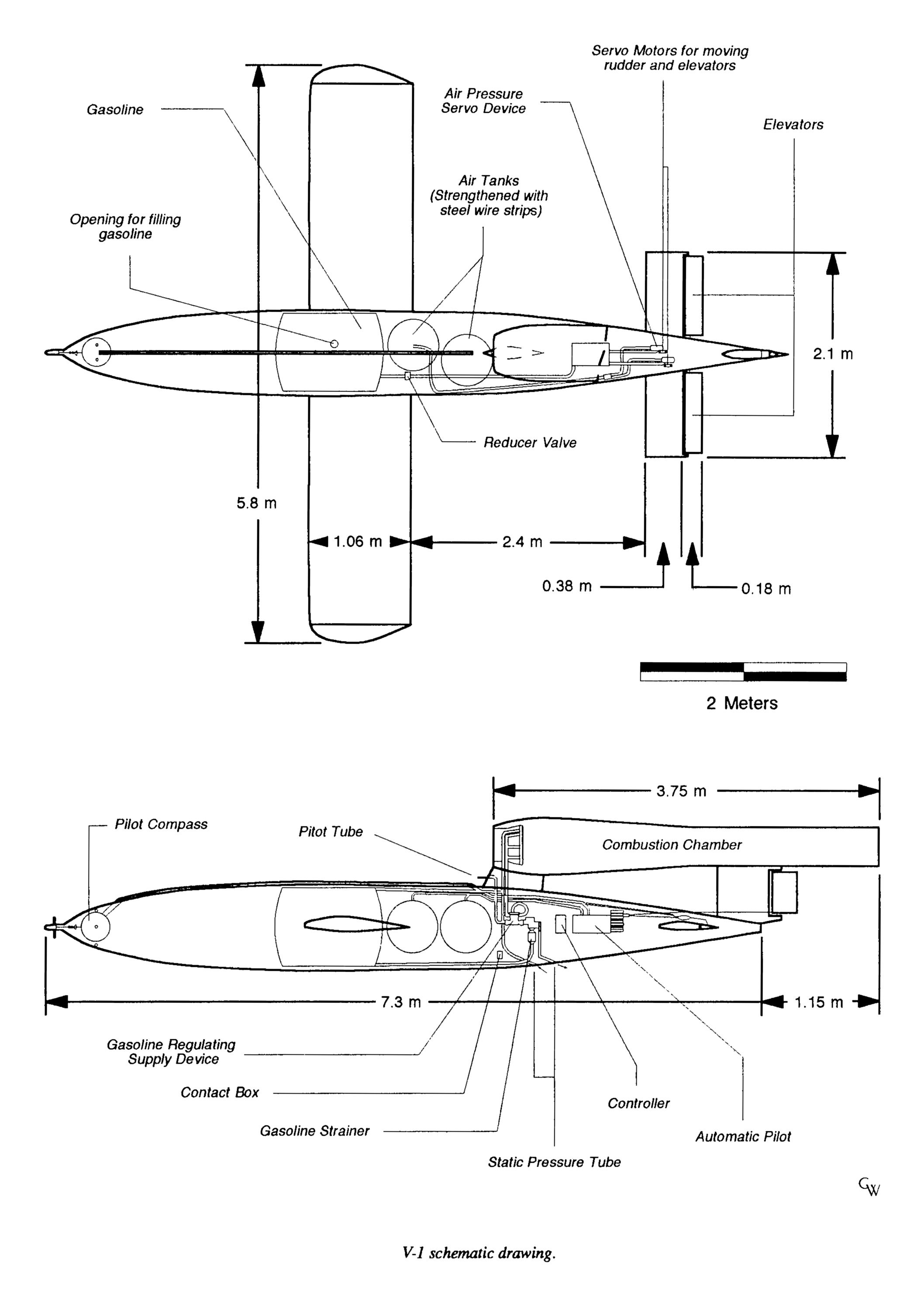This black and white diagram comprises two detailed schematic drawings labeled "V-1 Schematic Drawing," depicting what appears to be an airplane but could also be interpreted as a vehicle with aeronautical features. The schematics meticulously label various parts including gasoline tanks and openings for filling gasoline, air pressure systems, air tanks, motors, and elevators. It features boxes indicating measurements in meters, with arrows showing the lengths and directional orientations of different components. Detailed labels also point out a pilot compass, pilot tube, and a gasoline regulating device along with a gasoline strainer and the combustion chamber. Notably, there is a scale suggesting the objects are approximately 8 meters long, and a small logo with the letters "GW" is visible at the bottom right. The drawings lack any human figures and emphasize structural and functional details associated with the fuel and control systems of the aircraft.